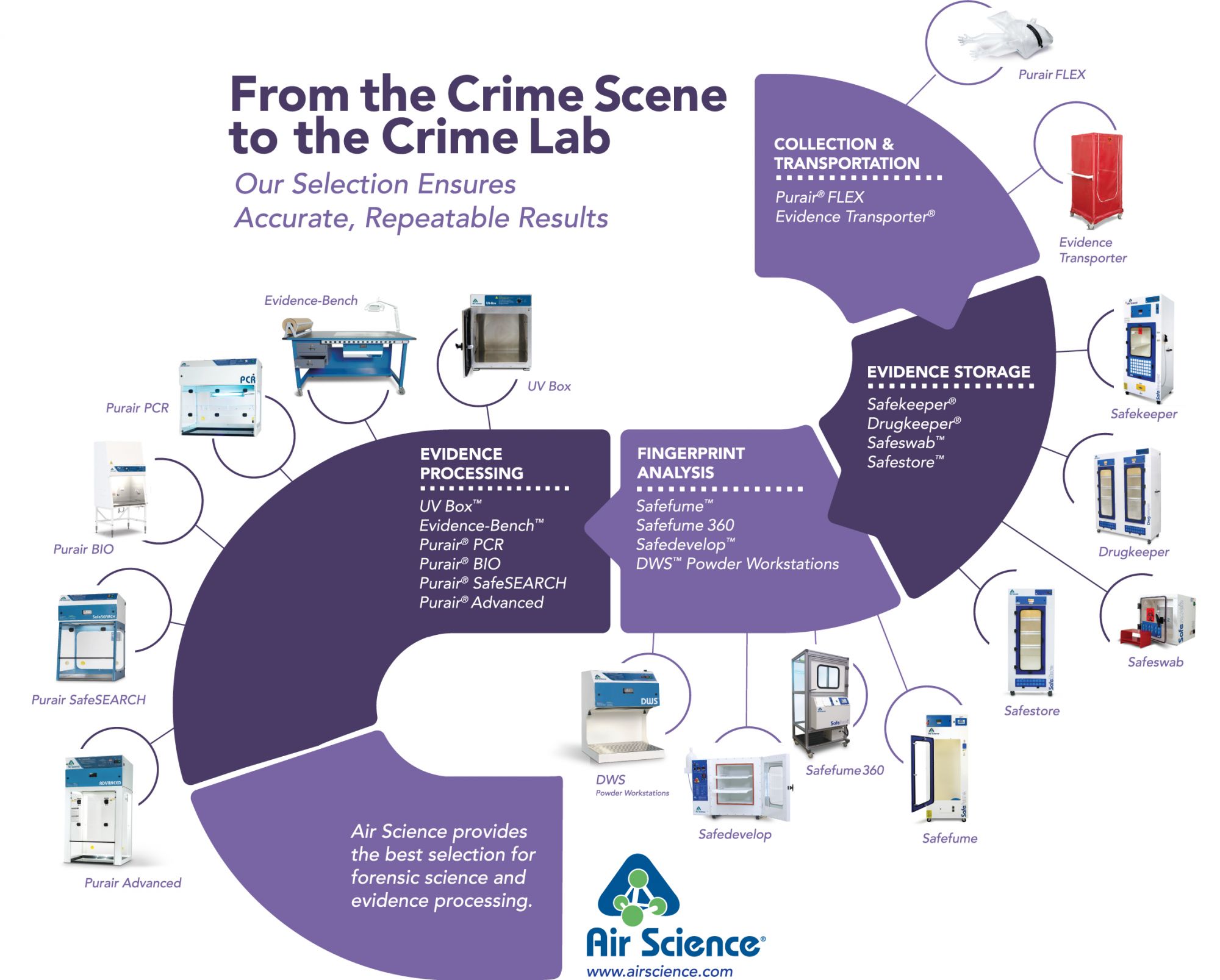This image, from Air Science, resembles a digital chart typically found in a book or a display. It is titled "From the Crime Scene to the Crime Lab: Our Selection Ensures Accurate, Repeatable Results," with the text prominently written in purple at the top left-hand side. The chart is organized in a pathway resembling a backward 'S' or the number '2', moving from the right down to the left. Adjacent to each section of the pathway are images of different pieces of crime lab equipment.

The chart categorizes the devices according to their use in various stages of an investigation and laboratory process:

- **Collection and Transportation:** Pure Air Flex Evidence Transporter.
- **Evidence Storage:** SafeKeeper, DrugKeeper, SafeSwap, SafeStore.
- **Fingerprint Analysis:** SafeFume, SafeFume 360, SafeDevelop, DWS Powered Workstations.
- **Evidence Processing:** UVBox, EvidenceBench, Pure Air PCR, Pure Air Bio, Pure Air SafeSearch, Pure Air Advanced.

The image utilizes a color scheme predominantly of purple and dark purple, with accents of red, white, blue, and yellow. At the bottom middle, the Air Science website, www.airscience.com, is displayed, emphasizing the company's commitment to providing quality forensic science and evidence processing equipment. The Air Science corporate logo, a tetrahedron with rainbows at the corners, is also featured.